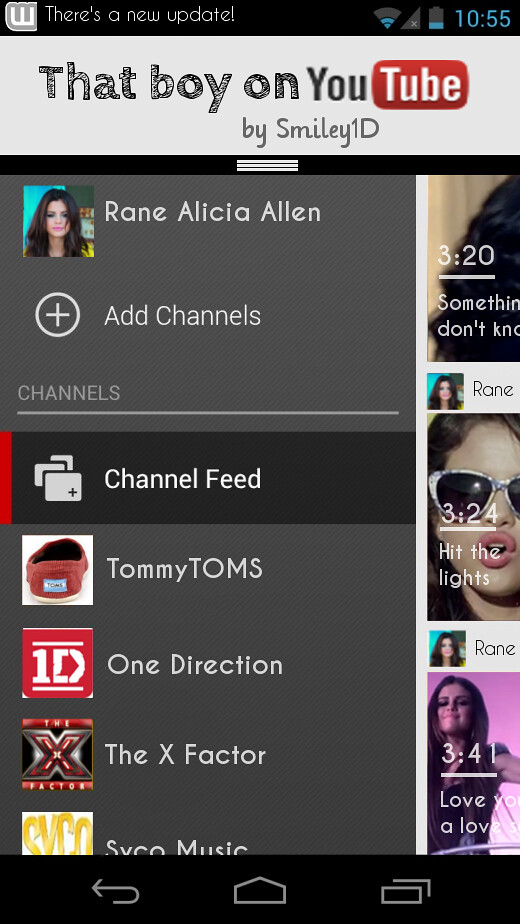The screenshot depicts a vertically oriented smartphone displaying a YouTube channel feed. At the top of the screen, a notification bar indicates a new update is available, shows that the phone is connected to Wi-Fi, and displays a low battery percentage with the time, 10:55. Below the notification bar, the screen displays the title "That Boy on YouTube" by Smiley1D in bold black lettering against a gray background. Next, there is an image of a girl accompanied by the name "Rainey Alicia Allen" and a plus symbol for adding channels. Underneath, a section titled "Channel Feed" lists various channels: "Tommy Tom's," "One Direction," "The X Factor," and "SVCO Music." To the right of these channels are song durations: "3:24" for "Hit the Lights," and "3:41" for "Love You." At the very bottom, three smartphone navigation icons confirm it is a mobile display. The overall image suggests the user is exploring music-related content on YouTube.